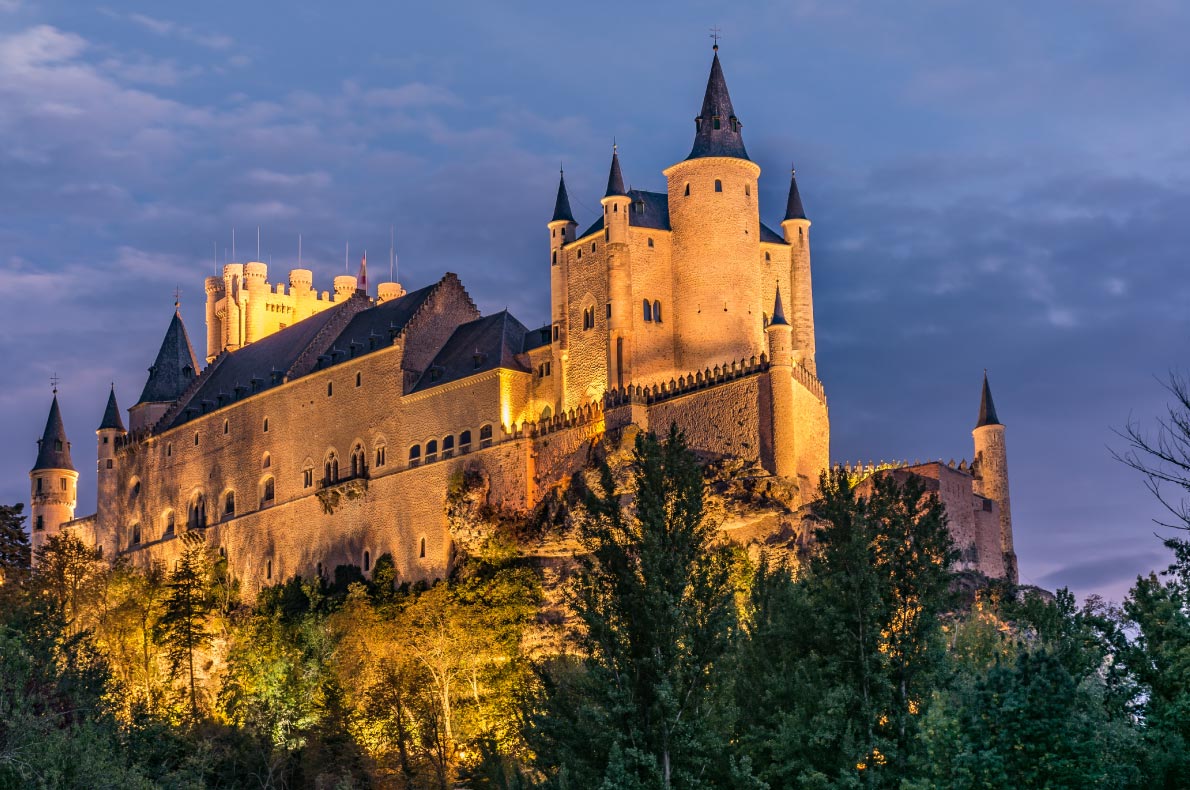In this mesmerizing photograph, a colossal castle commands attention as it majestically sits atop a picturesque hillside beside a serene body of water. The vast structure, featuring numerous spire-topped towers in dark gray, exudes an aura of strength and elegance with its off-white, almost vanilla-hued exterior. The surrounding landscape is adorned with a dense array of trees, accentuating the castle's imposing presence. The sky above is a mix of darkening clouds, suggesting that night is about to fall or rain is imminent. The castle is beautifully illuminated by numerous lights, casting a warm glow that highlights its intricate architecture. Small islands dot the distant water, enhancing the breathtaking scenery and making the entire scene look like a dreamlike destination, perfect for hosting many visitors. The overall grandeur suggests the castle boasts countless rooms, making it a formidable yet inviting edifice on the hillside.